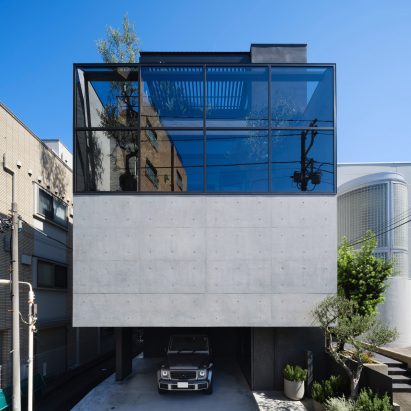The image captures an upscale, multi-story apartment building that resembles the architectural style often found in suburban areas like San Francisco. The structure is distinctively square-shaped, featuring a concrete base with a raised parking area where a high-end SUV is parked. Above the parking area, the building rises several stories, with the top floors characterized by large, blue-tinted, black-framed windows. These expansive windows offer a reflective view of an adjacent building, making it difficult to see inside clearly. 

Adjacent to the building, on the right side, a set of stairs leads up to the entrance, complemented by potted plants and other greenery, which contribute to the aesthetic appeal of the property. The sky in the background is a clear, light blue, indicating that the photo was taken during daytime. Surrounding the apartment are additional buildings to the left and right, adding to the urban, yet residential ambiance. There are no people visible in the image, adding a serene, almost still quality to the scene. Overall, the detailed architectural features and the carefully maintained greenery suggest a high-end, well-designed living space.